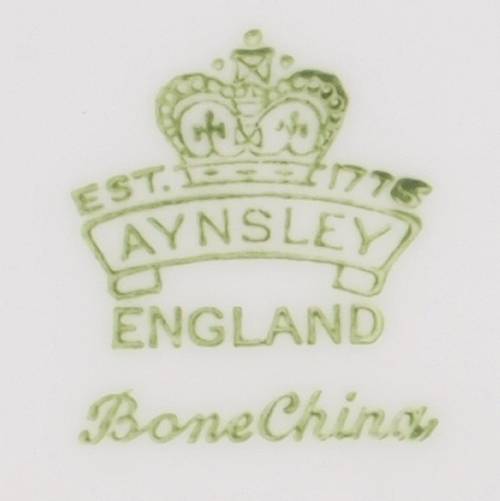The image is a square with an ivory or cream-colored background and features a detailed maker's mark or brand logo in a light green, natural-looking color. At the top of the logo is a crown adorned with dots and crosses. To the left of the crown it reads "EST." and to the right, "1775." Below the crown, the name "AYNSLEY" is written in all capital letters on a ribbon that curves upwards. Beneath "AYNSLEY," the word "ENGLAND" is printed in all capital letters, followed by the cursive words "Bone China" with both 'B' and 'C' capitalized. This finely detailed stamp is typical of marks found on the bottom of fine bone china, specifically from Ainslie, England, indicating the piece was established in 1775.